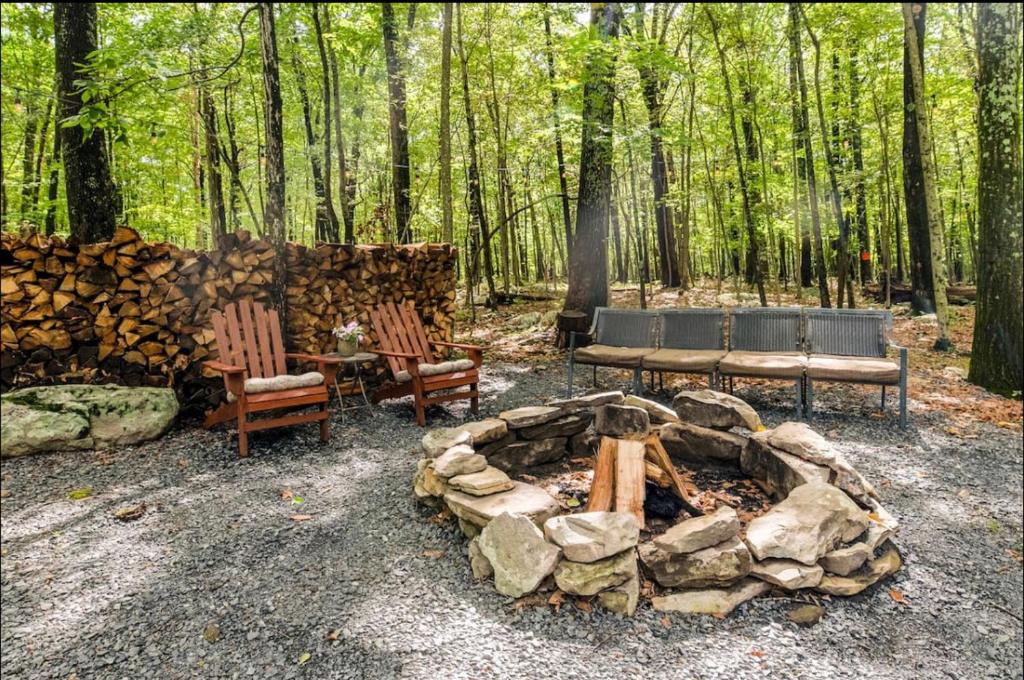The photograph captures a serene outdoor seating area amidst a forested setting. Central to the composition is a stone fire pit constructed from large, flat stones, with neatly stacked firewood standing upright in the middle. The fire pit sits in a gravel area with gray stones underfoot. Surrounding the fire pit are two distinctive types of seating arrangements. On the left, two brown Adirondack chairs with soft white cushions flank a small table adorned with a pretty pot of flowers, set against a backdrop of neatly stacked firewood. On the right, a row of four grayish-blue cushioned chairs lines the area, offering additional comfortable seating. The entire scene is enveloped by trees with slender trunks and light green leaves, reinforcing the sense of tranquility and seclusion, with a hint of rustic elegance, possibly indicating a well-maintained backyard recreational area. The color palette of red, brown, green, and gray enhances the natural beauty and warmth of the setting.